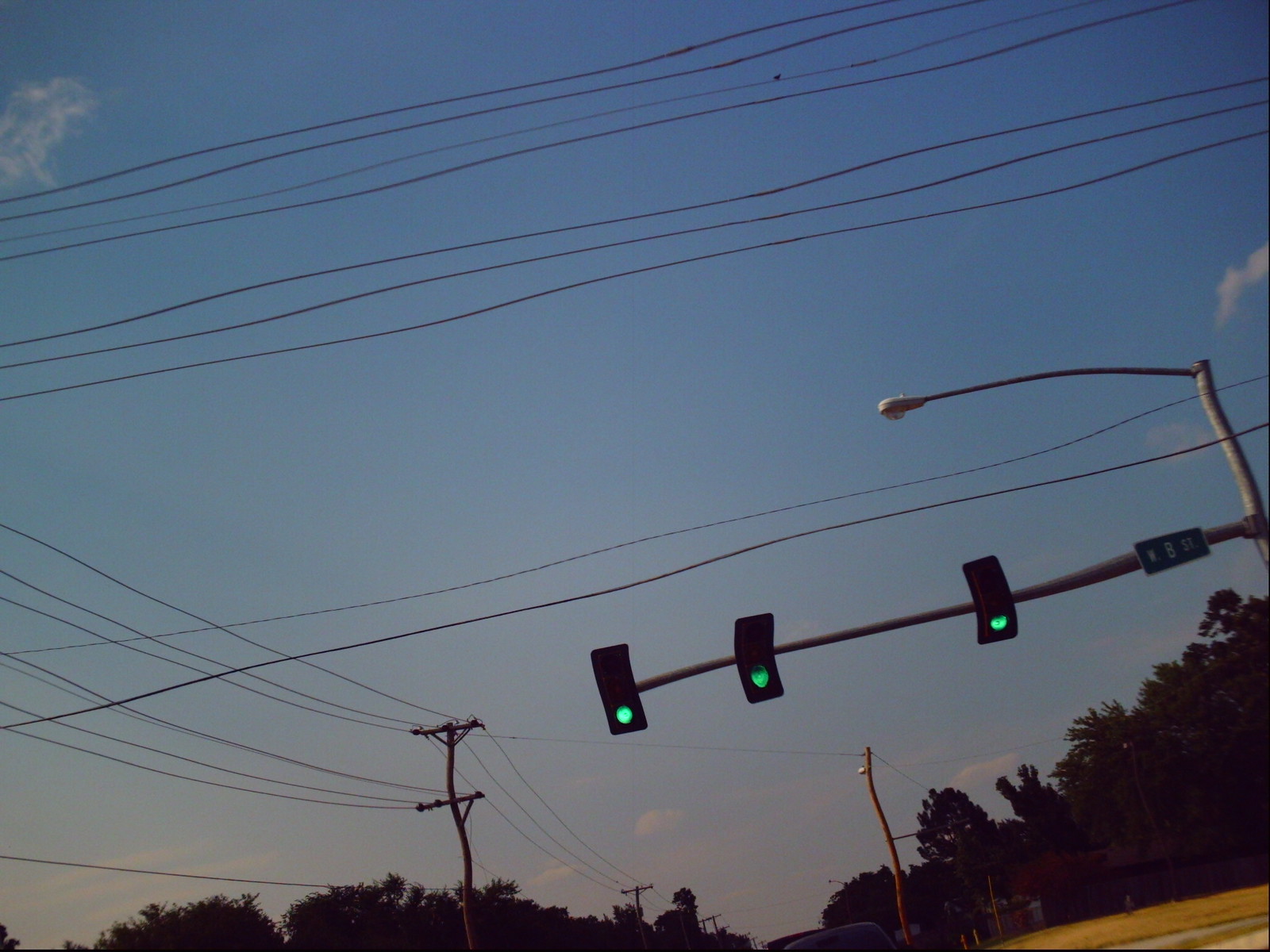The image displays a distorted view from what seems to be a dash cam, capturing a street scene dominated by a fairly clear sky transitioning from light blue to darkish blue hues towards the top. The sky is interspersed with faint patches of white clouds, particularly noticeable on the left and right edges of the picture. Central to the image is a tall, silver streetlight equipped with a light post that is off, indicating it's daytime. Attached to this pole is a green, rectangular street sign with white text that appears to read "8th Street" or "B Street." Below this sign are three vertically aligned traffic lights, all showing green, yet noticeably warped and curving due to what seems like an editing effect or a space-time disturbance, giving the scene a surreal appearance. In the background, lush green trees fill the lower portion of the image. Also prominent are brown wooden power poles with black electrical lines stretching vertically and horizontally across the scene, further adding to the warped and wobbly look of the objects in the picture.